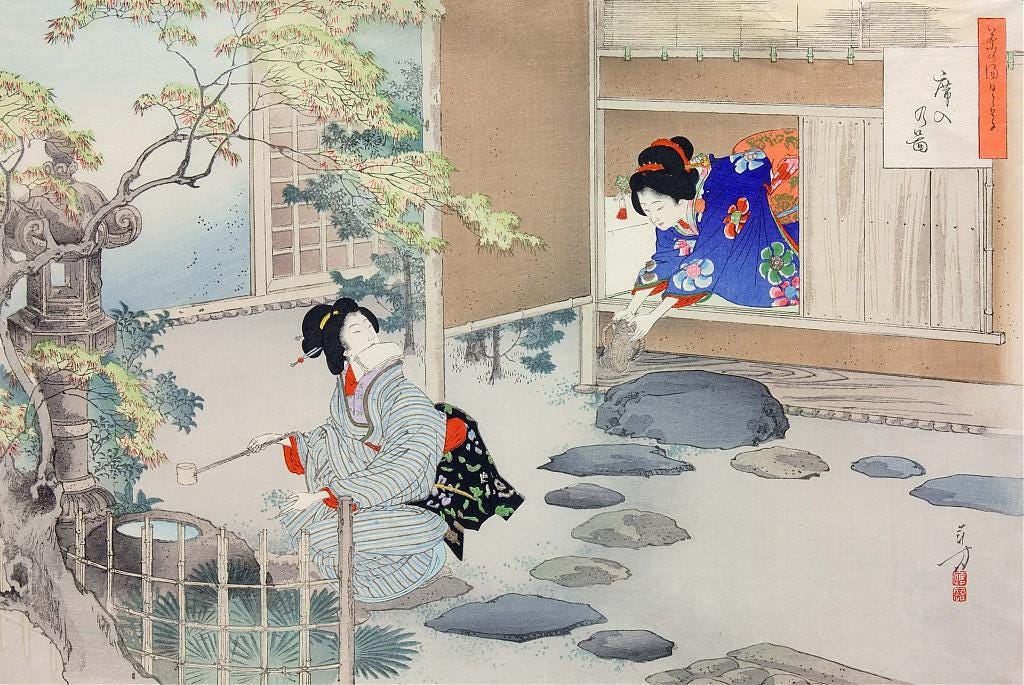This detailed Japanese-style woodblock print features two geishas in traditional kimonos within a serene, garden setting. On the right side of the scene, a woman is positioned inside a building, peering out of a wooden-slatted window with distinctive wooden curtains. Her hair is elegantly tied up with red decorations, and she's donned in a blue dress adorned with a vibrant array of flowers - red, blue, green, and pink. She is extending her hands outside the window, seemingly scooping or washing something in the water below, surrounded by rocks and elements of a Japanese garden. Above her, there is Japanese writing on both a tan square and an orange rectangle.

To the left, another geisha is in a kneeling position near a well-like water source, holding a bamboo water scoop. Her head is turned towards the other woman, her hair wrapped in a yellow bun. She wears a layered ensemble, featuring a white undergarment, a blue and white striped robe with red accents on the sleeves and back, and possibly an object strapped to her back. Behind her is a fence and verdant green plants, with a tree extending its branches towards the top left side of the image. Additional intricate details include a small black object with green and gray squiggle patterns and a tiny statue beneath the tree, as well as small squiggly drawings on the lower right side of the print.